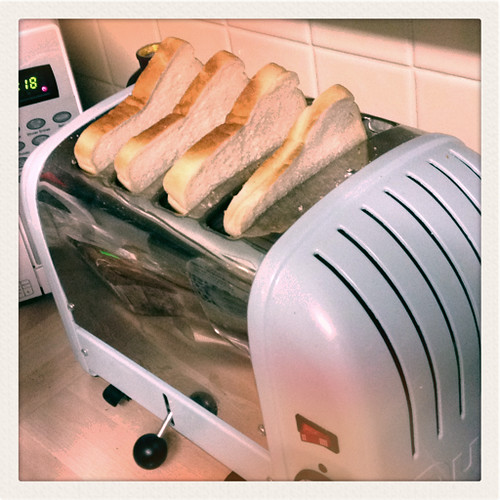This is a close-up, color-filtered photograph of a retro-style four-slice toaster. The image is framed in a light gray border and features the toaster prominently positioned on a beige wooden countertop. The toaster has a distinctive design with a silver metal body and white or light blue plastic ends, although the true colors are obscured due to a color filter. Four slices of white bread are inserted in each of the four slots, angling slightly to the left, and they are not yet toasted. The toaster includes a black knob at the bottom, likely for raising or lowering the bread, and a red switch on the right side. To the left of the toaster, partially visible, is a white microwave oven with a silver exterior and gray buttons. The microwave display reads "18," indicating time, and is set against a white tiled wall with white grout.